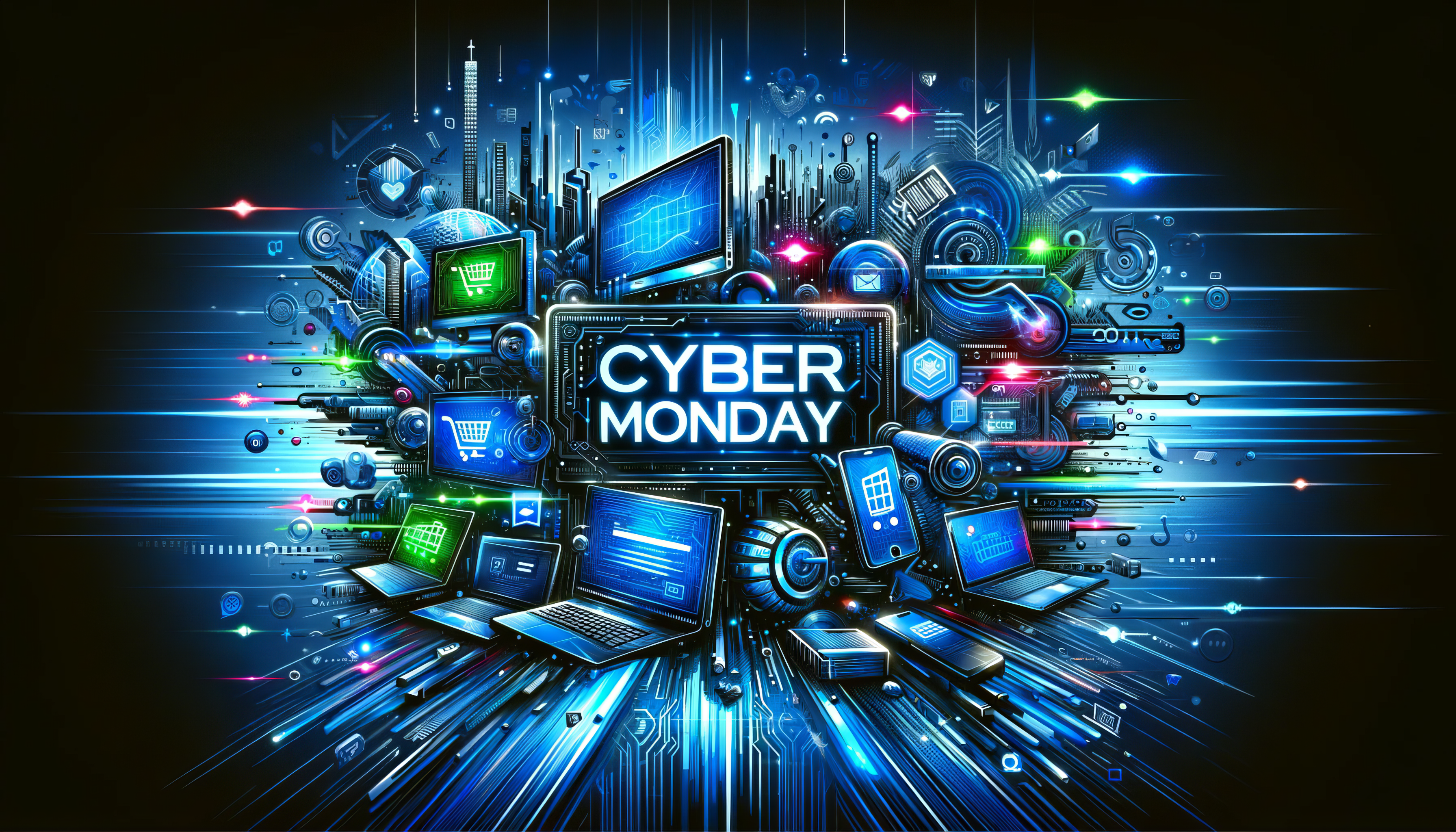The image is a vibrant, computer-generated artwork illustrating Cyber Monday, set against a very dark, almost black background. At its center, glowing white letters spell out "Cyber Monday," surrounded by a chaotic array of electronic gadgets, including computer monitors, laptops, cell phones, and TVs, their screens flickering with electric blues, greens, pinks, and light grays. Star-like colorful designs radiate around the devices, creating a starburst effect that emphasizes the bustling energy of the scene. The overall aesthetic is futuristic, with a stark contrast between the dark background and the bright, luminous colors, capturing the frenetic essence of the shopping event.